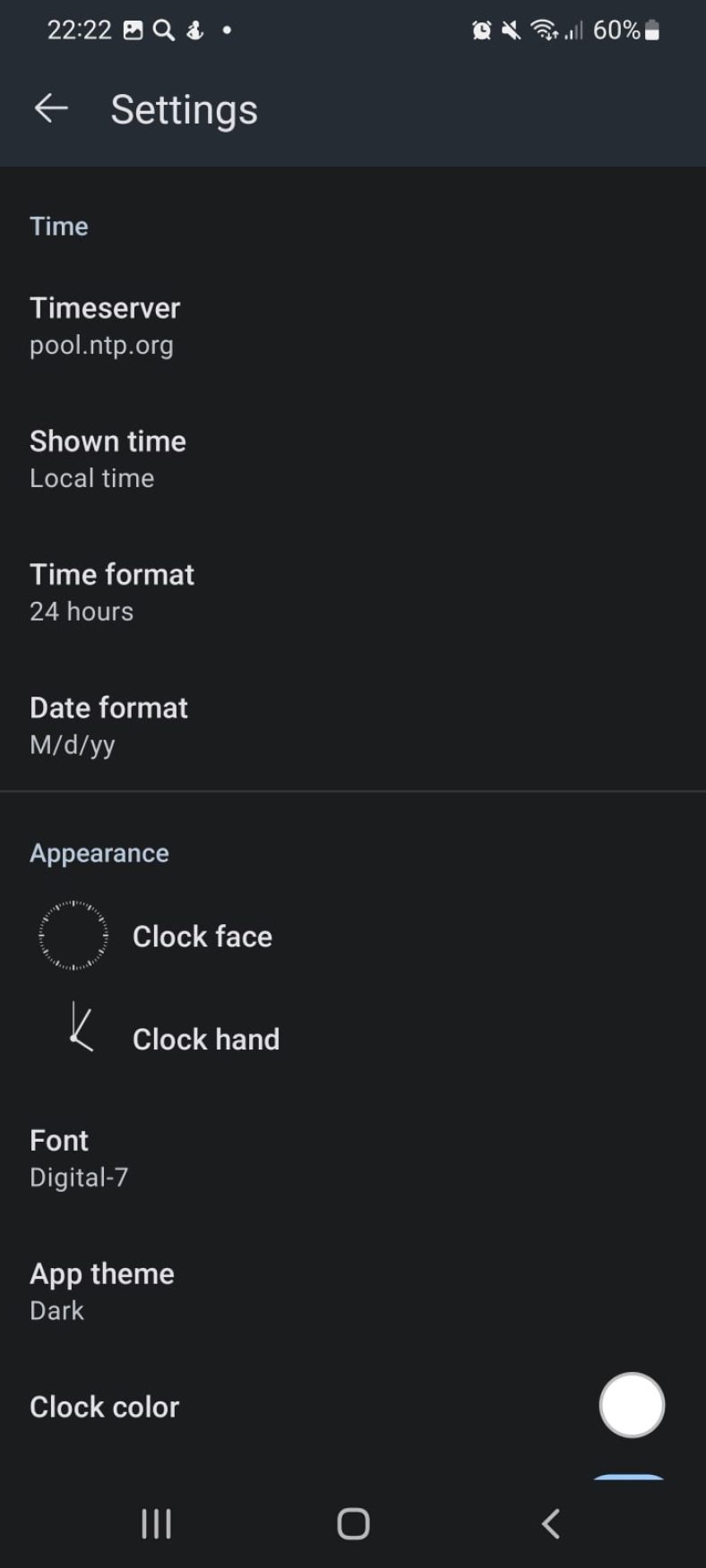In this screenshot captured from a smartphone—judging by the screen size and overall layout—we observe a dark gray bezel framing the display. The top of the bezel prominently displays the time "2222" in bold white text, indicating military time. There's a notification alerting the user of the captured screenshot, depicted as a white square featuring a black sun above black mountains, accompanied by white icons of a magnifying glass, a running figure, and a white circle suggesting additional notifications.

Adjacent to this notification on the right-hand side, we notice the system clock along with several status icons: a muted sound symbol (a speaker with a line through it), a full Wi-Fi signal, and a cell phone signal showing two out of four bars. Beside these icons, "60%" is indicated next to a battery icon displaying a little over half charge.

On the bottom part of the bezel, there's a white arrow pointing left with the label "Settings." The screen transitions from black to white text, presenting various settings in gray and white fonts. It starts with "Time" in gray followed by "Time Saver" in bold white. Subsequent options include "pool.ntp.org" in gray, and other settings such as "Local time" and "Time format: 24 hours", each accompanied by gray descriptions.

Advancing through the options, we encounter "Date format: MM/DD/YY" and "Appearance" both in gray. A visual of a dotted circle resembling a speedometer or compass is also displayed here, followed by "Clock Face," "Clock Hand," and "Font: Digital-7" each labeled in bold white. Additional settings detail "App Theme: Dark" and "Clock Color" in bold white, with a white circle featuring a blue underline beside it.

Finally, at the bottom bezel of the smartphone, there are three navigation options: three horizontal lines for selecting settings or different windows, a rounded square for minimizing apps, and a back arrow pointing left.